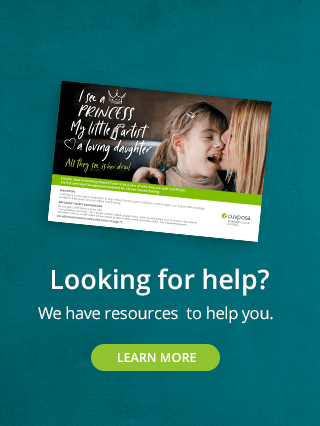The image features a dark blue background with a central, tilted photograph. In the photo, a young girl with pigtails, a silver barrette, and bangs appears with her eyes closed and mouth open in a joyful smile. A woman with long blonde hair, facing left, is tenderly kissing the girl's cheek. Text overlaid on the image reads, "I see a princess, my little artist, a loving daughter. All they see is her," followed by an illegible word. Below the photo, there is a line of text too small to read clearly. Further down, the blue banner background contains a message in white letters: "Looking for help? We have resources to help you." At the very bottom, a green oblong button with the words "Learn more" is displayed in white text. The image is oriented vertically, and does not contain any animals, birds, fish, plants, flowers, trees, buildings, or automobiles.